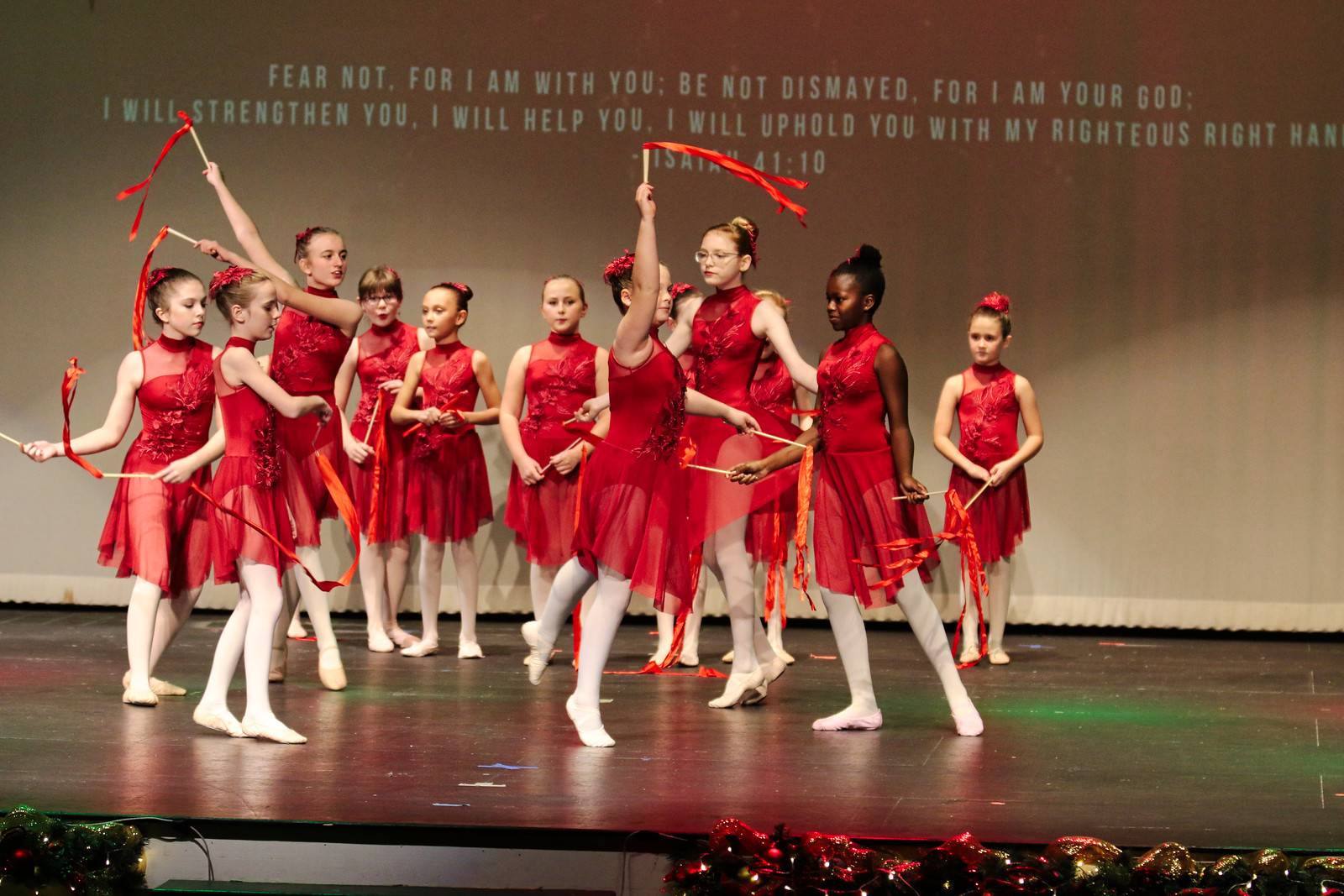This color photograph captures approximately a dozen young girls performing a dance on a stage. Each girl is dressed in a ballerina-like costume that features red flowers on the front, a sheer red skirt, white tights, and small red bows in their hair. They are all holding sticks with red streamers, captured in various dance poses and movements. The stage is adorned with artificial greenery and multicolored string lights around its border. Projected onto the white curtain behind them is a Bible verse: "Fear not, for I am with you. Be not dismayed, for I am your God. I will strengthen you. I will help you. I will uphold you with my righteous right hand. Isaiah 41:10."